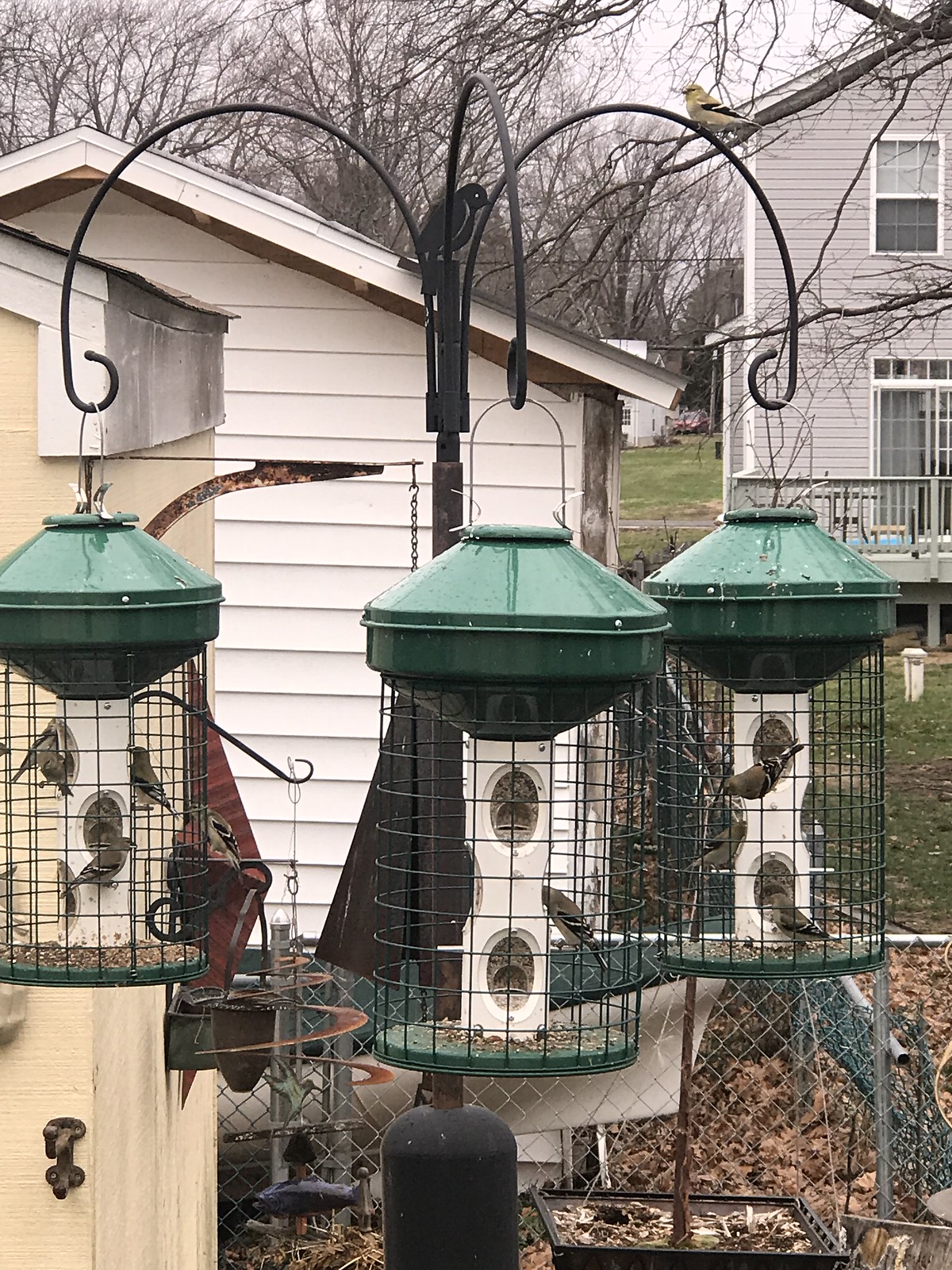This detailed colour photograph, captured in portrait orientation, showcases an outdoor scene in a garden featuring several bird feeders prominently positioned in the bottom half of the image. The focal point is a cluster of three green, cylindrical bird feeders with wire constructions designed to deter squirrels while allowing small birds to access the bird seed inside. The feeders hang from a triple shepherd's hook and are surrounded by various birds enjoying the food.

In the background, the setting includes a small shed with white horizontal panelling and a pitched roof located towards the middle left of the image. Additionally, the backdrop features the light grey side of a residential house with vertical railings on a back porch, alongside a sliding door that opens onto a grey-painted deck. 

A chain-link fence extends from behind the shed, stopping at its edge, and the white, shingled roof of what appears to be a detached garage or another part of the residence is visible. The scene suggests it is either late fall or winter, with some trees void of leaves, dry straw-like material on the ground beneath the feeders, and patches of dark green grass. The overall composition conveys a tranquil backyard habitat tailored for birdwatching.